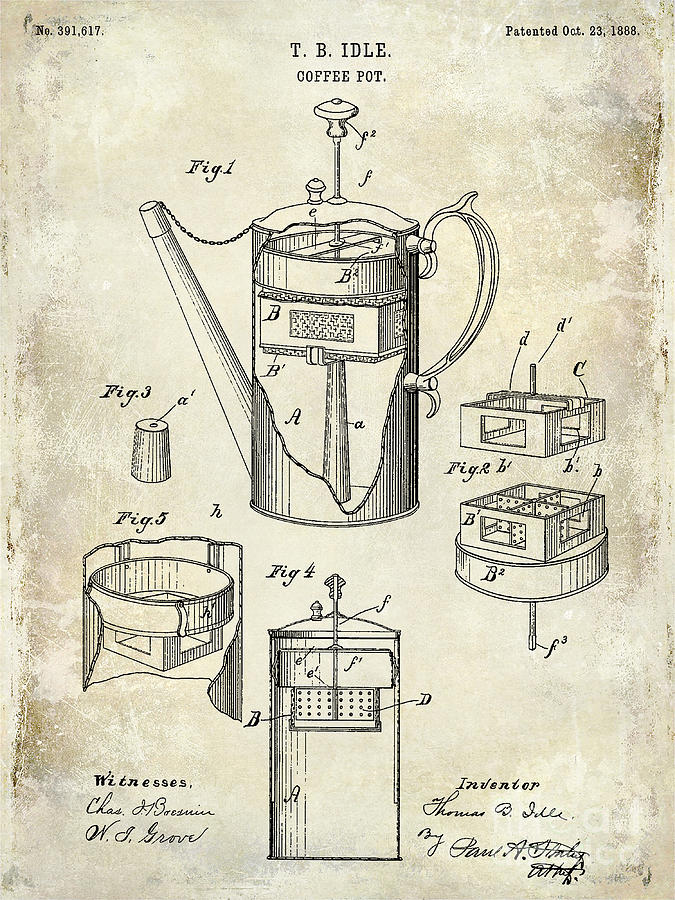This image is a highly detailed vintage black and white line-art illustration of an original coffee pot patent dated October 23rd, 1888. The illustration is set on aged, oxidized brownish parchment paper. At the top center, the text reads "T.B. Eitel Coffee Pot," and in the upper right corner, "Patented October 23rd, 1888." The upper left corner displays the patent number "391,617."

The central image is a profile view of the coffee pot, showing intricate details of its design. The coffee pot features a long, diagonally angled spout connected to its bottom and a handle riveted to the side. Inside, the drawing highlights various components, including a cylindrical part running through the center and a circle component that appears to be part of the coffee brewing mechanism. Each part is labeled with blowout labels that include letters (e.g., uppercase 'B' and 'A') and notations like lowercase 'f' to the second power.

Beneath the central image, additional illustrations labeled as figure 1, figure 2, figure 3, figure 4, and figure 5 showcase different angles and details of the coffee pot, including its interior components and detachable parts. The bottom section of the illustration features the words "Witnesses" and "Inventor," each followed by signatures. There is also evidence of a crossed-out signature among the inventor's names.

Overall, the illustration is a meticulous and historically rich depiction of a patented coffee pot, showcasing both its outer design and internal mechanisms.